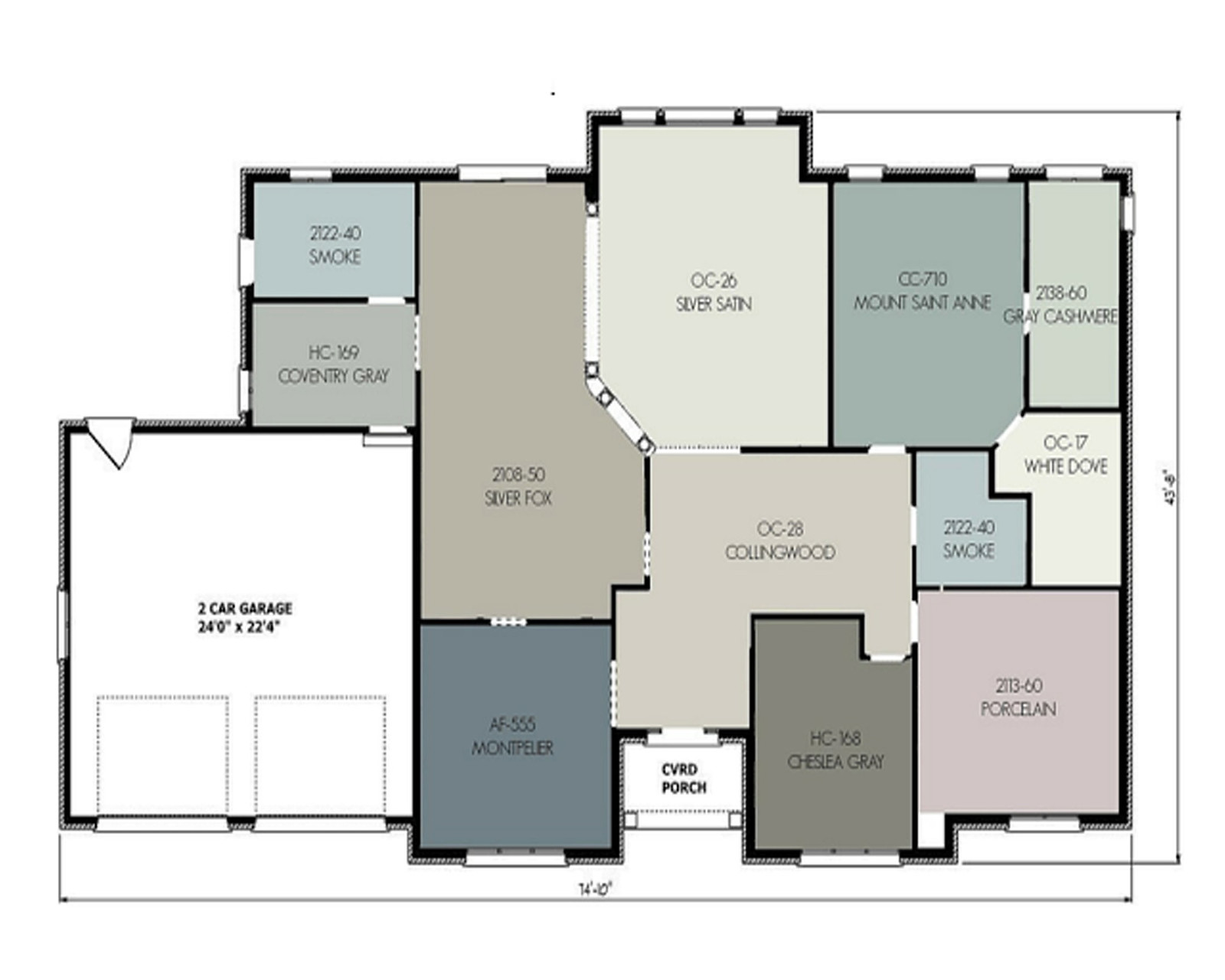This image showcases a detailed floor plan, highlighting the paint color scheme for various rooms, although the specific purposes of the rooms are not labeled. On the far left, there is a spacious two-car garage measuring 24x22, which notably doesn’t have a paint color assigned. The floor plan indicates a diverse palette of colors for the different areas, including Smoke, Covington Gray, Silver Fox, Montpelier, Silver Satin, Mt. St. Anne, Gray Cashmere, and White Dove. Among these, Porcelain stands out as a very pale pink, while Collingwood offers a tan hue. The different shades of gray—Montpelier, Smoke, Covington Gray, and others—dominate the color scheme, giving the interior a sophisticated, monochromatic look. Despite the lack of room labels, the visual display of hues such as Chelsea Gray and Mt. St. Anne helps visualize the interior aesthetic of the house.